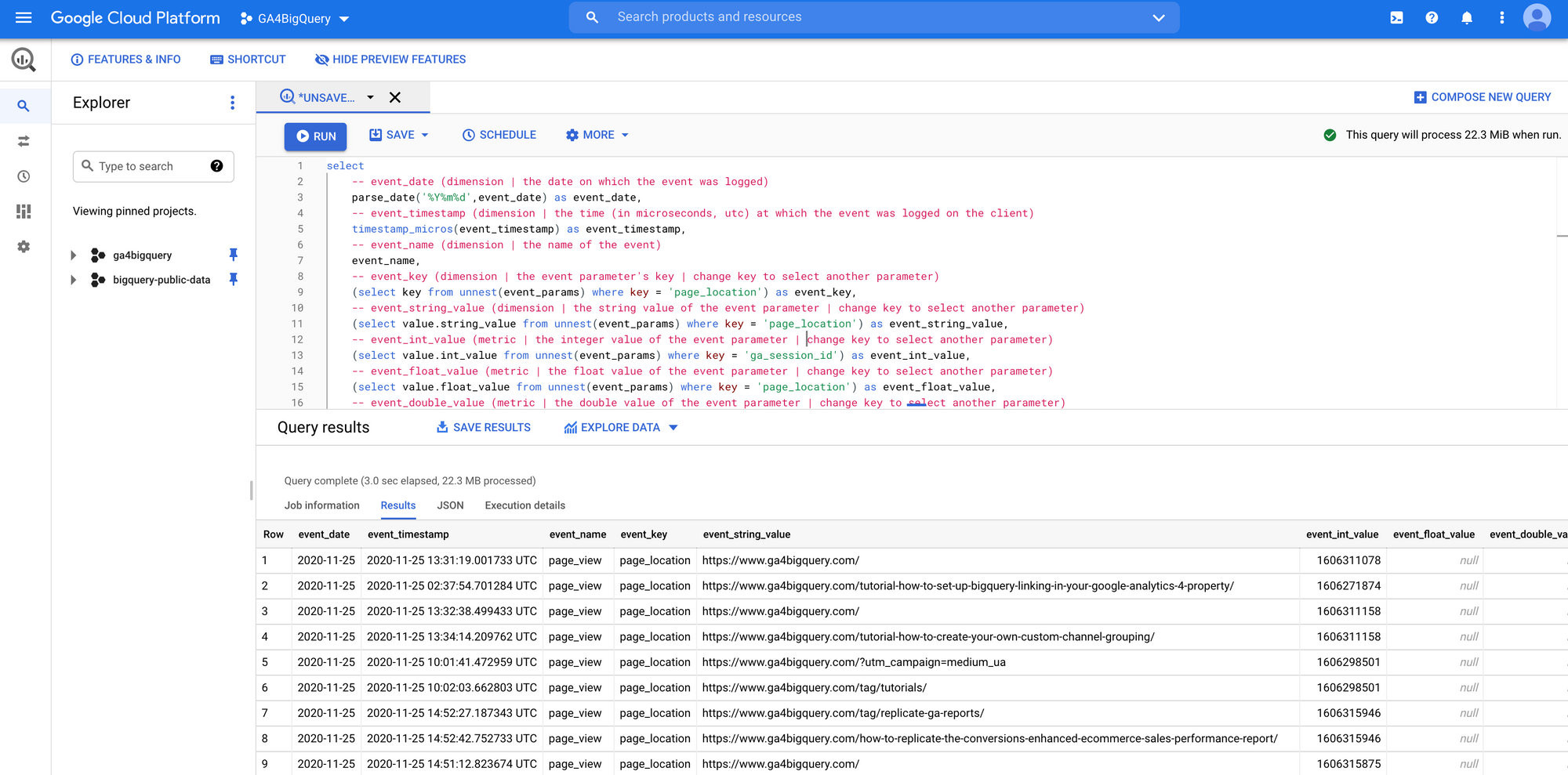The image depicts a Google Cloud interface where a script is being executed within the GA4 BigQuery project. At the top left, the Google Cloud logo is prominently displayed in white, adjacent to a drop-down menu labeled "GA4 BigQuery," marked by a triangular arrangement of three dots. On the far left, a three-line menu icon is visible above a search bar labeled "Search products and resources," accompanied by a drop-down option. Directly beneath the search bar are icons for feature info, shortcuts, hiding the preview feature, and an explore tab with a search field.

To the right of this sidebar, the main content area shows an active script execution. The interface highlights that the user is currently on the "Run" tab, with additional buttons for "Save," "Schedule," and "More" to manage the script. A notification indicates that the query will process 22.3 units, with the script involving approximately 16 commands. The scripting area displays syntax-highlighted text in pink, green, and blue.

Below the script area, there's a section for "Query results" featuring options to save results and explore data further. This is followed by detailed tabs for job information, results in JSON format, and execution specifics. The current view is set to "Results," presenting a table with columns for event date, event time, name, event key, string value, event int value, and float value.